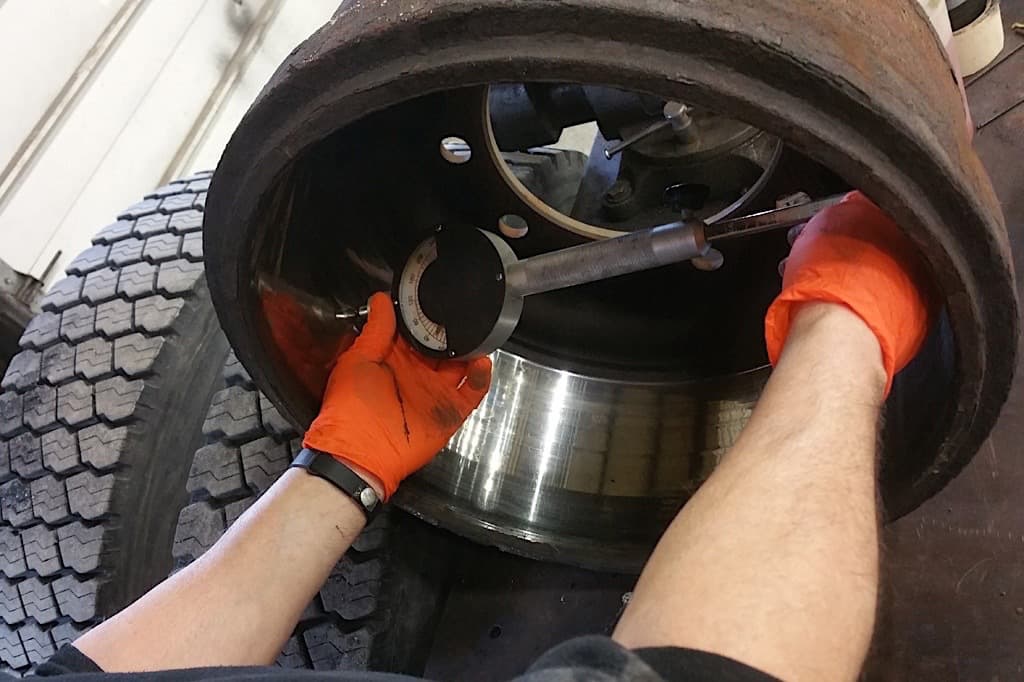In this detailed photograph, a white Caucasian individual, identifiable by a smooth black wristband on their left wrist and distinctive orange gloves, is engaged in automotive work. The focal point of the image is a rusted gray metal barrel-like structure situated centrally, which appears to be a heavily used car part. Prominently displayed is a pressure gauge, featuring a white face with black lettering and a red dial, affixed to a grayish metal pipe. The gauge is pressed inside an inner compartment likely associated with the vehicle's wheel assembly, discernible by its silver inner surface transitioning to a blackened back end and rusted brown outer edges. To the left of the barrel, a black treaded tire with a white wall rim is visible, suggesting proximity to other car parts. The workspace is punctuated by a dark gray floor extending to the far right, providing a stark contrast to the various automotive components scattered around.